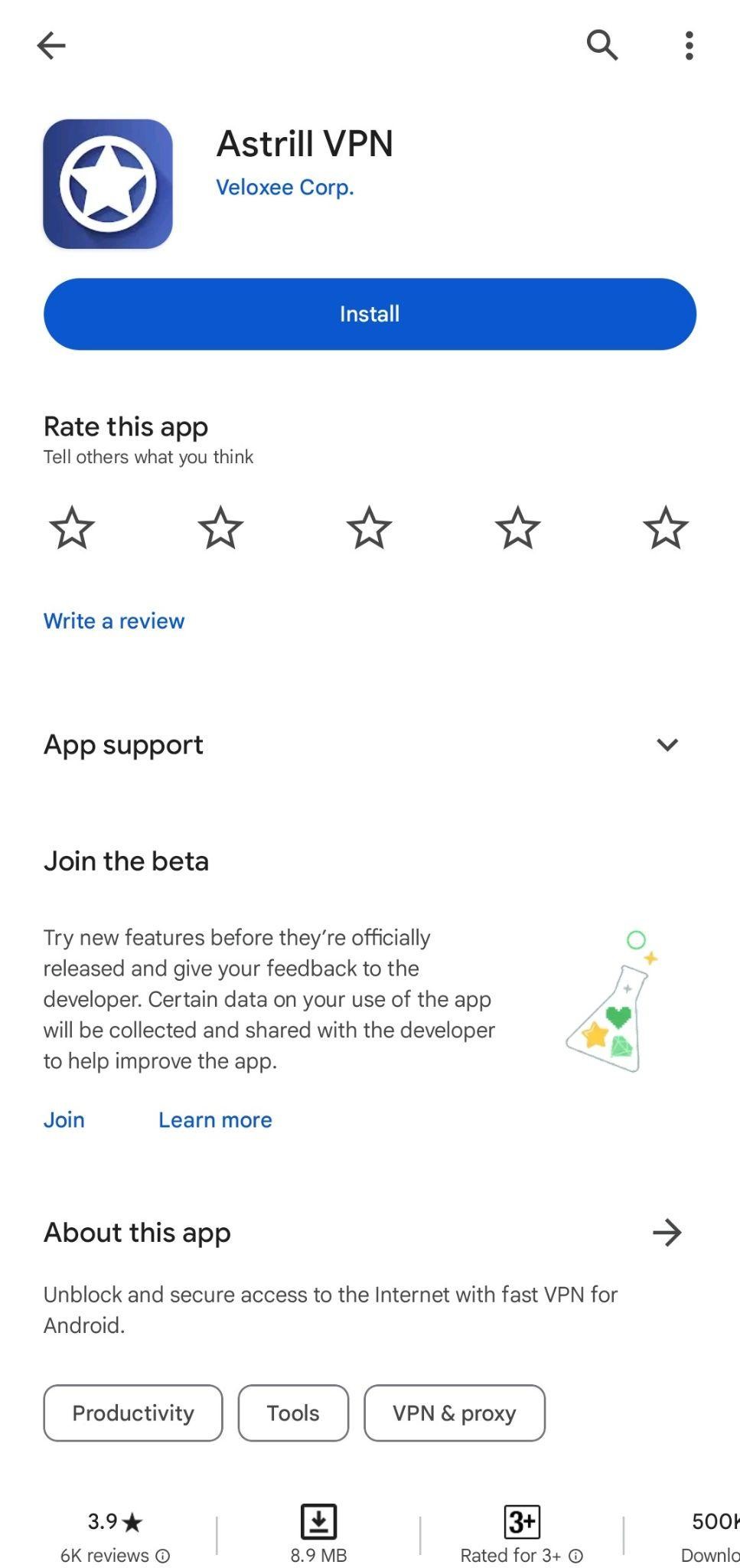In the screenshot, the user is exploring the app store to find more information about an app called "Astral VPN" developed by Biloxi Corp. The app's logo features a blue box with a design resembling a Captain America star. At the top of the screen, there is a back arrow indicating that the user can navigate to the previous page.

Detailed information about the app is displayed, including an option to install it. Users are encouraged to rate the app and share their opinions, as indicated by the presence of five clickable stars for rating (none of which are currently selected) and a hyperlink inviting users to write a review. An additional link is available for app support.

The app store entry mentions an option to join a beta program, allowing users to test new features before their official release and provide feedback to the developer. It notes that certain data on app usage will be collected and shared with the developer to aid in the app's improvement. A science beaker icon with various elements emerging from it visually represents the beta program, accompanied by hyperlinks to join the beta or learn more about it.

Under the "About This App" section, a brief description states: "Unblock and secure access to the internet with a fast VPN for Android." The app is categorized under Productivity Tools, VPN, and Proxy.

Astral VPN has a rating of 3.9 stars based on 6,000 reviews. The app's size is listed as 8.9 MB, and it is rated suitable for users aged 3 and up. The app has over 500,000 downloads, though the exact number is slightly obscured in the screenshot.